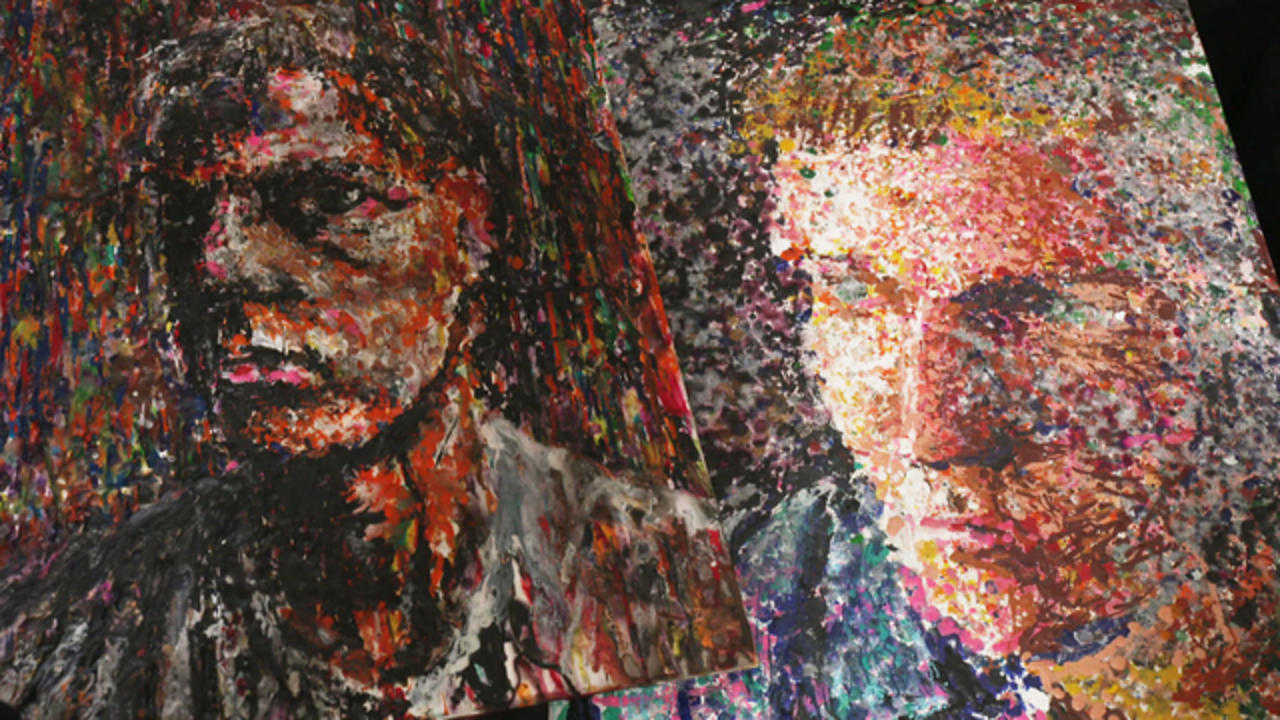The image features two distinct paintings, which, upon close inspection, resemble a pointillist technique similar to Monet's style, composed entirely of tiny dots of paint that come together to form detailed portraits from a distance. The left painting is of an African man, characterized by a more naïve artistic approach with harsh, contrasting colors such as dark reds and blacks that create a stark, shadowy effect. His skin is depicted in very dark brown, almost onyx-like tones, with red accents, and his large, dark brown eyes appear prominently. His bottom lip is fuller with hints of red and pink, while the top lip is thinner with a bit of black above it. He is wearing a gray shirt. This portrait stands on top of another canvas.

Beneath, a more realistic painting portrays a Caucasian man whose features are rendered with blended, vibrant colors that appear softer and more natural. The strokes here, though equally chaotic, create smoother transitions between colors, mainly browns and skin tones that suggest a lifelike quality. His blonde hair contrasts vividly against his light skin, and his bluish-green eyes and soft pink lips are clearly defined. He is dressed in a brighter blue shirt.

Together, these paintings exhibit the fascinating dichotomy between abstract pointillist detail and realism, capturing the essence and contrast of two different subjects in terms of color and technique.